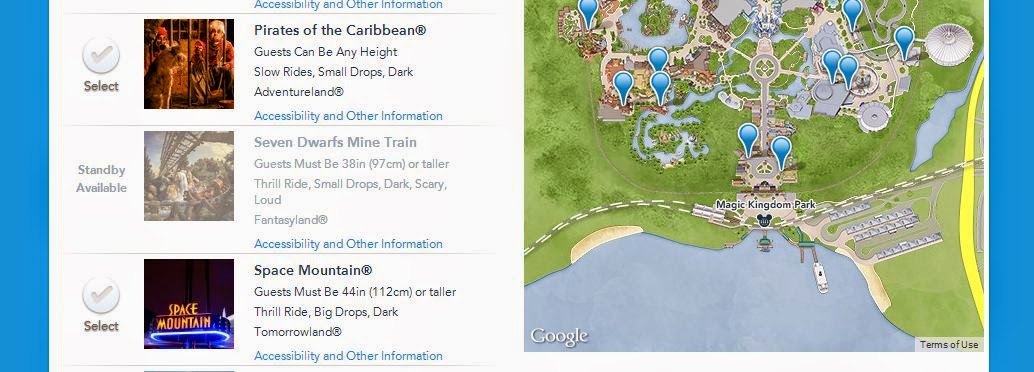The image is divided into two main sections: the right-hand side features a detailed map, while the left showcases a series of images and descriptions related to various attractions.

### Right-Hand Side:
The map displayed on the right is predominantly dark green, interspersed with areas of tan, brown, lighter tan, and yellow. A multitude of dark blue pins with white borders mark various locations. A gray band with white dashes runs through the map, bordered by a dark blue section. Additionally, a white ship icon is present on the map. At the bottom left corner, the word "Google" is displayed in white text. On the right, there’s a gray rectangle containing the black text "Terms of Use". A yellow band stretches across the map, flanked by dark blue rectangular bands on both the left and right sides.

### Left-Hand Side:
Below is a detailed description of each image and the associated text on the left-hand side:

1. **Lion Cage Image**: 
   - The first image shows a person crouching in front of a lion's cage, with the lion looking directly at him. The lion features a brown and tan coat. In the background, several individuals appear to be wearing red turbans. The person crouching has white hair, a red shirt, and black pants. 
   - Text to the right in bold black reads: "Pirates in the Caribbean".
   - Additional descriptive text in regular black reads: "Guests can be any height, slow rides, small drops, dark adventure land". 
   - An "R" inside a black circle follows.
   - Hyperlinked blue text at the top and bottom reads: "Accessibility and Other Information".
   - A circle on the left features a 3D effect with a black border and bluish-white interior, containing a dark gray checkmark. Below it, bold black text reads: "Select".

2. **Roller Coaster Image**: 
   - The next image depicts a faded-out roller coaster, appearing brown with green trees in the background, indicating it is not available for selection.
   - To the left, in faded gray text, it says: "Stand By Available".
   - To the right, in faded gray text, it says: "Seven Dwarf Mine Train: Guests must be 38 inches (97 cm) or taller, thrill ride, small drops, dark, scary, loud".
   - The text concludes with "Fantasyland" and an "R" inside a black circle.
   - Hyperlinked text at the bottom reads: "Accessibility and Other Information".

3. **Space Mountain Sign Image**: 
   - The final close-up image features an orange and yellow sign that reads "Space Mountain".
   - The signage is held by an oval-shaped neon blue and purple LED display.
   - Another circle on the left is similarly colored to the previous one, with a black checkmark.
   - To the right, in bold black text, it says: "Space Mountain", followed by an "R" inside a bold black circle.
   - Regular black text below states: "Guests must be 44 inches (112 cm) or taller, Thrill Ride, Big Drops, Dark, Tomorrowland".
   - Hyperlinked blue text at the bottom reads: "Availability and Other Information".

This cleaned-up and detailed caption provides a comprehensive description of the entire image, capturing the intricate details and textual information presented.